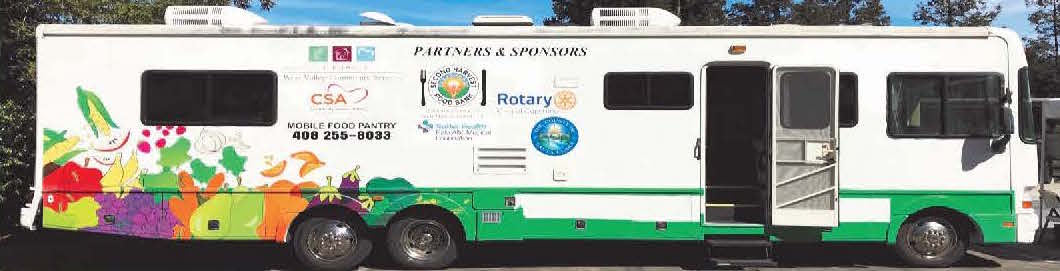The image depicts a very large, rectangular, white bus that was once a motorhome, now repurposed as a mobile food pantry. The bus has a unique three-wheel configuration with one set of wheels in the front and two sets in the back. Adorned with a vivid green strip along the bottom, it features detailed illustrations of various fruits and vegetables with faces, including corn, apples, grapes, carrots, and eggplants, especially towards the rear above the wheel. The side of the bus prominently displays multiple logos and text related to its function and sponsors. Key phrases such as "Partners and Sponsors," "Rotary Mobile Food Pantry," "CSA Second Harvest Food Bank," and a contact number "408-255-8033" are clearly visible. The image, set against a bright blue sky on a sunny day with trees in the background, captures the mobile pantry parked, showcasing its role in providing food in parking lots. The bus's door is open, emphasizing its accessibility for those in need.